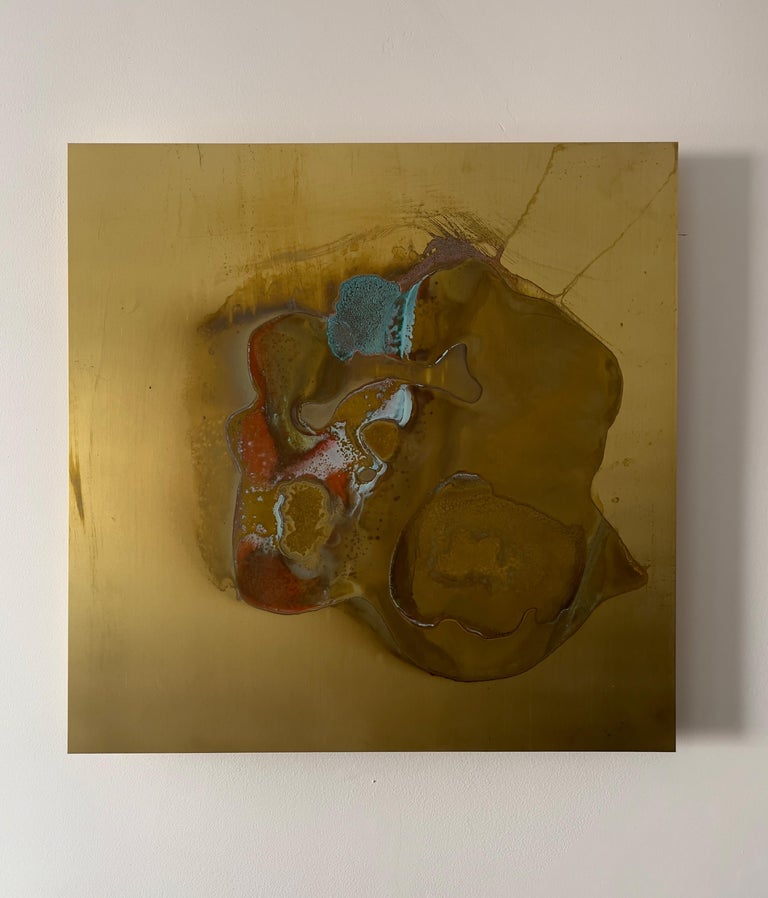The image features a predominantly brown, abstract piece of art set against a yellow background. The artwork, which appears to be a square-shaped painting, suggests the look of a rock partially submerged in water. The rock-like form transitions between wet and dry textures, with the part sticking out appearing dry and located in the bottom right section. The submerged sections exhibit a darker blue hue, contrasting with the creamy, whitish-blue tones of the exposed parts. Additional colors, such as reddish and grayish tones, are visible around the bottom left corner and the top left corner, which also shows traces of blue. A light source to the left casts shadows across the painting, enhancing the darker yellow tones, particularly towards the bottom right corner. The abstract nature of the piece gives it a splotchy appearance, reminiscent of a cross-section of an animal, while maintaining an overall brown and tan palette with splashes of red and blue amidst the shadowed and highlighted areas.